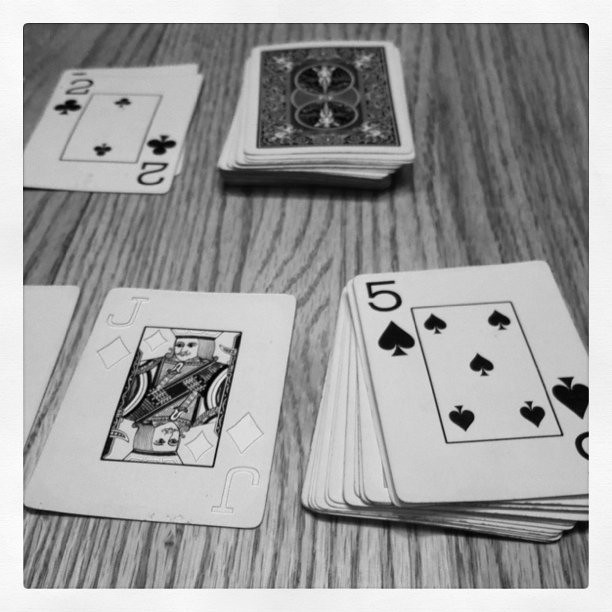In this black-and-white image, a variety of playing cards are meticulously arranged on a wooden surface, likely a table. The central focus is a neatly stacked deck of Bicycle playing cards positioned slightly above the center of the image. These cards feature the iconic Bicycle design with twin angels in opposing circular positions, surrounded by a spiral pattern.

To the left of this main stack, two cards overlap each other. Below and to the right, another smaller stack of face-up cards can be seen, with the top card being the Five of Spades. Adjacent to this stack, a single card, the Jack of Diamonds, rests on the left.

Additionally, slightly above and to the left of the central stack, there are two face-up cards. One of these cards, fully visible, is the Two of Clubs, while the identity of the other remains obscured. 

The wooden surface underlying all the cards features distinct vertical grain lines, adding texture and depth to the monochromatic composition.